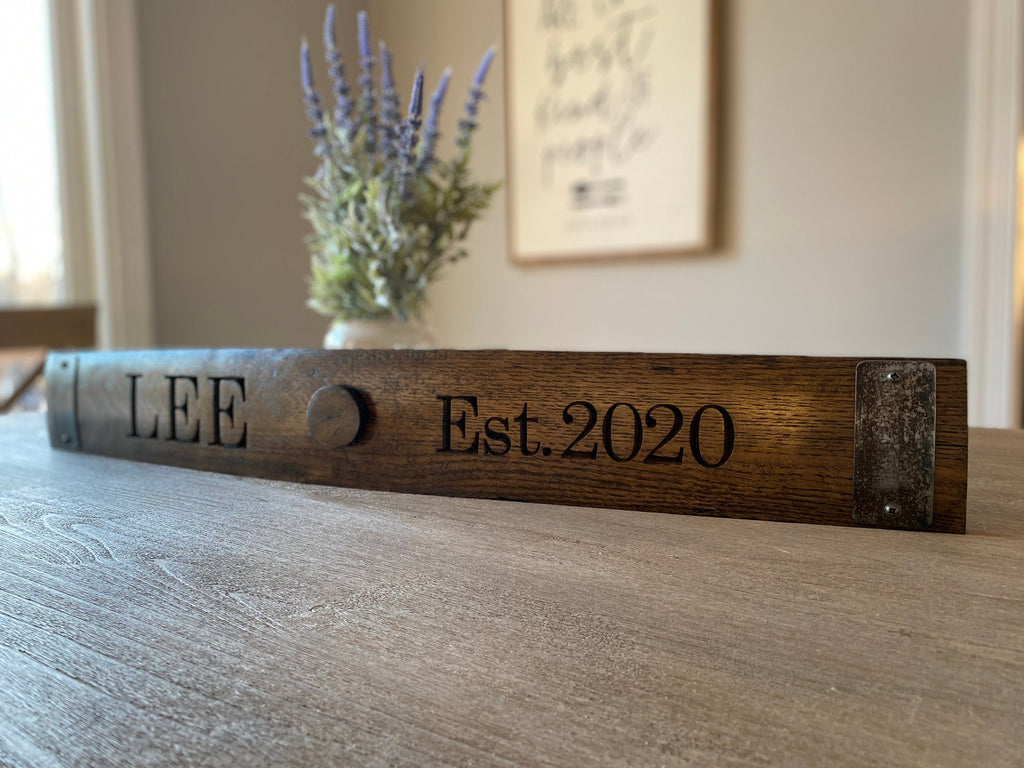This is a detailed color photograph of an indoor setting illuminated by natural light streaming in from a partially visible window on the left. Dominating the center of the image is a rustic, long wooden placket on a light wooden table. The placket is engraved with the name "LEE" in capital letters towards the left, followed by "EST. 2020" to the right. The surface of the wood is rough-hewn, adding to its rustic charm. Adjacent to the placket, a white vase filled with tall, purple lavender flowers adds a touch of elegance. In the blurred background, a framed artwork with cursive writing is faintly visible, hanging on gray walls. No people, animals, or mechanical objects are present in the photograph, focusing the viewer's attention on the serene and artfully arranged indoor scene.